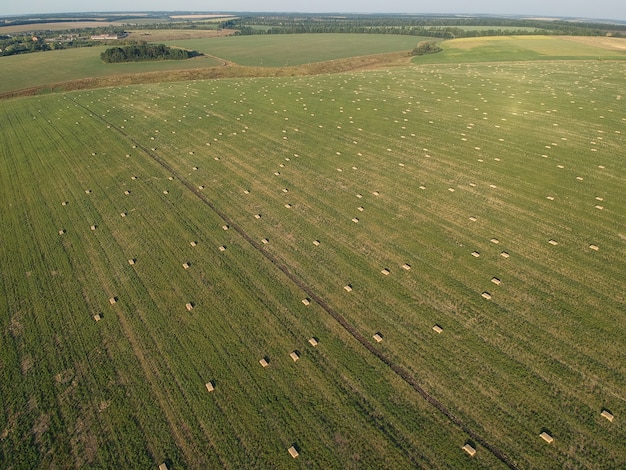This is an aerial view of a vast green field, possibly farmland, depicted from a height that allows visibility far into the distance, yet close enough to discern details. The landscape is characterized by neat, linear patterns, indicative of plowed land. Scattered throughout the expansive field are numerous rectangular or square shapes which, upon close observation, appear to be bales of hay, their cream or light yellow color contrasting against the green. The field spans a considerable area, estimated between 20 acres to 10 miles squared, suggesting it’s a sizable piece of farmland. There are no visible houses or buildings within the immediate vicinity of the field itself. The sky above appears partly cloudy, casting a diffused light over the scene without intense sunshine. Off in the distance, beyond the open field, groups of tall trees and possibly small structures – either small farms or cement blocks – can be seen, hinting at the edges of the farmland where possibly businesses or houses may reside.